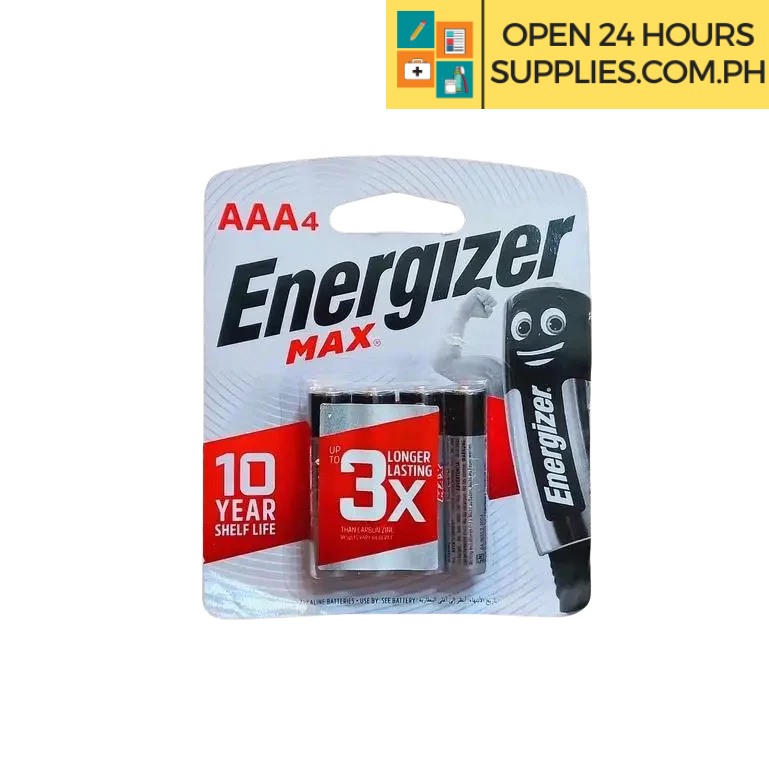This image showcases a package of batteries in a highly detailed manner. In the upper right-hand corner, there is a rectangular section featuring a yellow background with a black vertical line on the left side. To the immediate left of this line, there are four icons: a pencil, a case with a cross symbol on the front, hygiene items, and a paper form. To the right of the black line, it reads "Open 24 Hours, supplies.com.ph."

Dominating the center of the image is a package containing four AAA Energizer Max batteries. The packaging highlights that these batteries offer a 10-year shelf life and are three times longer lasting. To the right side of the battery package, there is a cartoon image of a battery with expressive eyes and a wide smile. The cartoon battery's right arm is extended outward and bent at the elbow, with the forearm pointing upwards and the fist clenched, giving a lively and energetic impression.